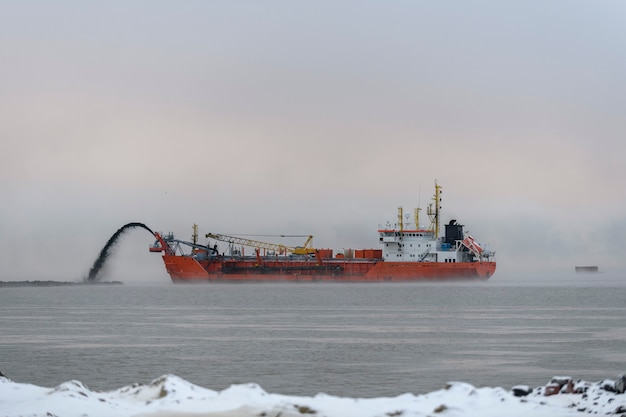This photograph captures a scene of a large, bright orange industrial ship positioned in icy waters on a dreary, overcast day. The ship, likely in the Arctic, stands out due to its vibrant hue and prominent features. At the ship's center, a yellow crane lays on its side, while three yellow towers rise above a white superstructure where the control center is likely located. The vessel is ejecting a stream of black liquid from its left side, arcing into the murky gray waters below. The scene is framed by a snowy, rocky shoreline in the foreground, and a vast expanse of ocean stretches between the land and the distant ship. The sky is a hazy blend of pink, blue, and gray tones, contributing to the overall misty and foggy appearance of the setting.